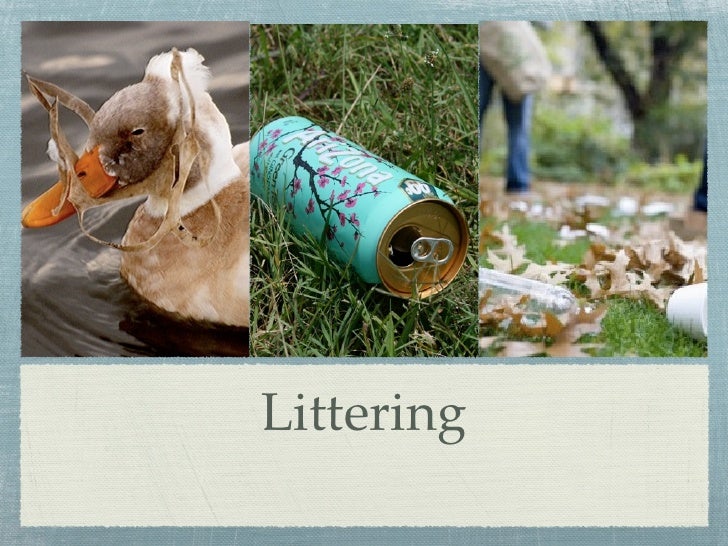The image is a wide, rectangular infographic likely used in a presentation to address the issue of littering. It is bordered by a light green outline. The top two-thirds of the infographic is divided into three equal vertical panels, each containing a photo illustrating different instances of littering. The first panel shows a gray duckling with a yellow beak, swimming in dark green water, entangled with a piece of plastic or paper around its head. The middle panel features a discarded light blue Arizona tea can lying on green grass, its label clearly visible. The third panel depicts a park scene with various pieces of trash, including styrofoam cups and plastic bottles, scattered on the ground. In this panel, you can also see the legs of a person in the background, seemingly engaged in cleanup efforts. The bottom third of the infographic is a wide, horizontal section in a tan color, with the word "littering" prominently centered in green lettering. This visually straightforward but impactful design is evidently used to emphasize the detrimental effects of littering on the environment.